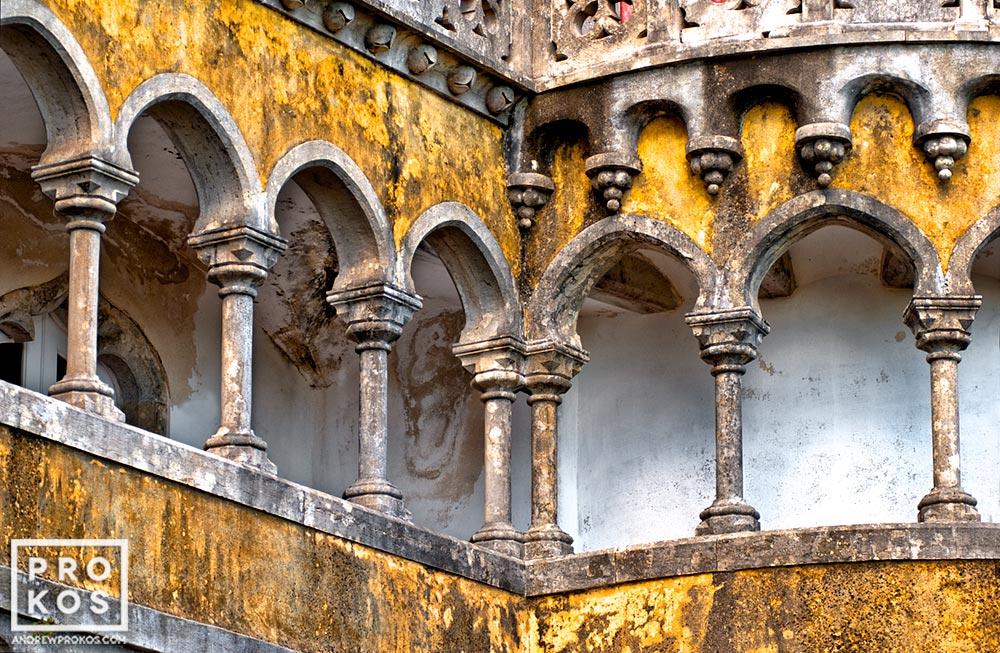This photograph captures a historical stone structure characterized by its ancient, weathered architecture. The focal point includes seven pillars that support a series of arches. These arches span both horizontally and above one another, creating a layered, intricate design. The stone is heavily stained and weathered, showing discoloration in shades of gray, yellow, and brown, with the remnants of golden paint adding to its aged appearance. Water stains mark the back wall, suggesting a long history exposed to the elements. The overall look of the building hints at Roman architectural influences, possibly an ancient aqueduct or a segment of Roman baths. The photograph, credited to Andrew Prokos (as indicated by the watermark "Prokos, AndrewProkos.com" on the bottom left), offers a view from the ground up, emphasizing the grandeur and historical significance of the ruins.